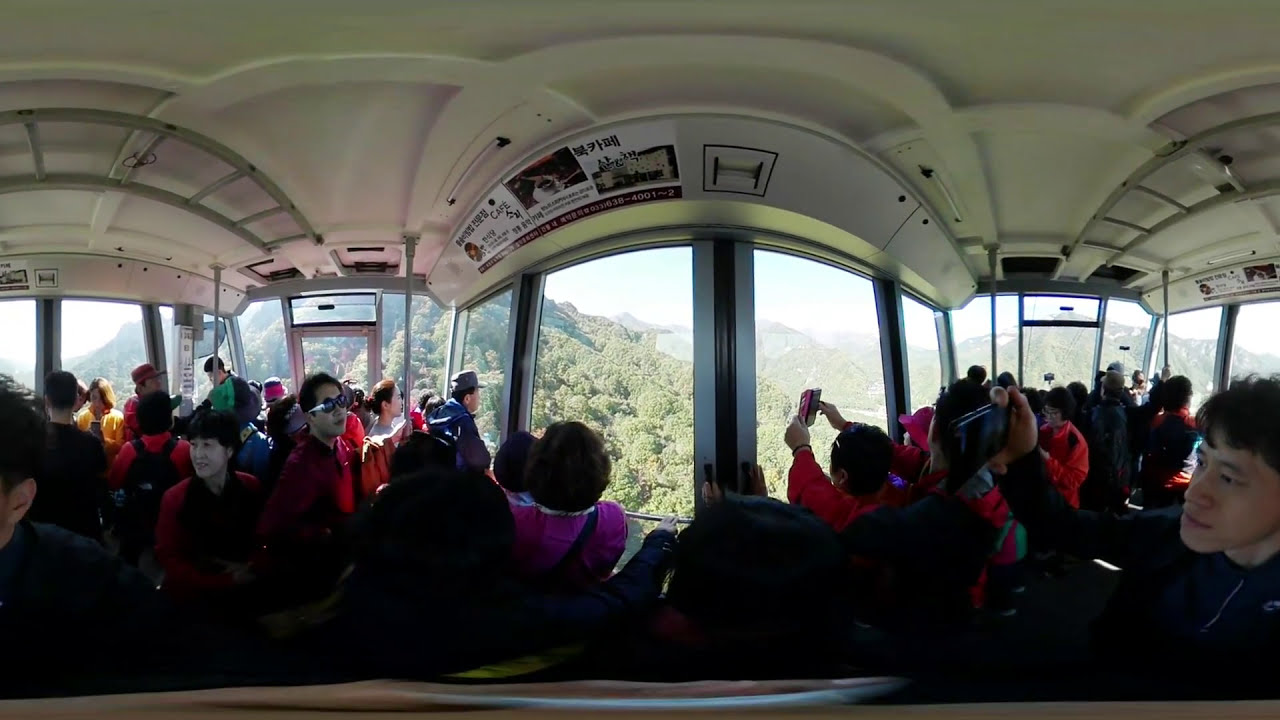The image depicts the interior of a 360-degree glass-enclosed gondola lift, possibly located in China or Japan, as it traverses a mountainous, tree-covered landscape. The gondola, roughly the size of a bus, is filled with tourists of various ages, predominantly of Asian descent, who are visibly engrossed in the scenic views outside the large floor-to-ceiling windows. Many of the passengers are holding up their cell phones to capture photographs of the verdant surroundings. Clear signage and advertisements, written in what appears to be an East Asian language - likely Chinese or Japanese - are visible on the ceiling of the gondola. The panoramic view provided by the image includes an expansive and lush mountainside bathed in bright sunlight, suggesting a clear, pleasant day. The fisheye effect from the 360-degree photo adds to the immersive experience, emphasizing the gondola's elevation and the vast, picturesque nature below.